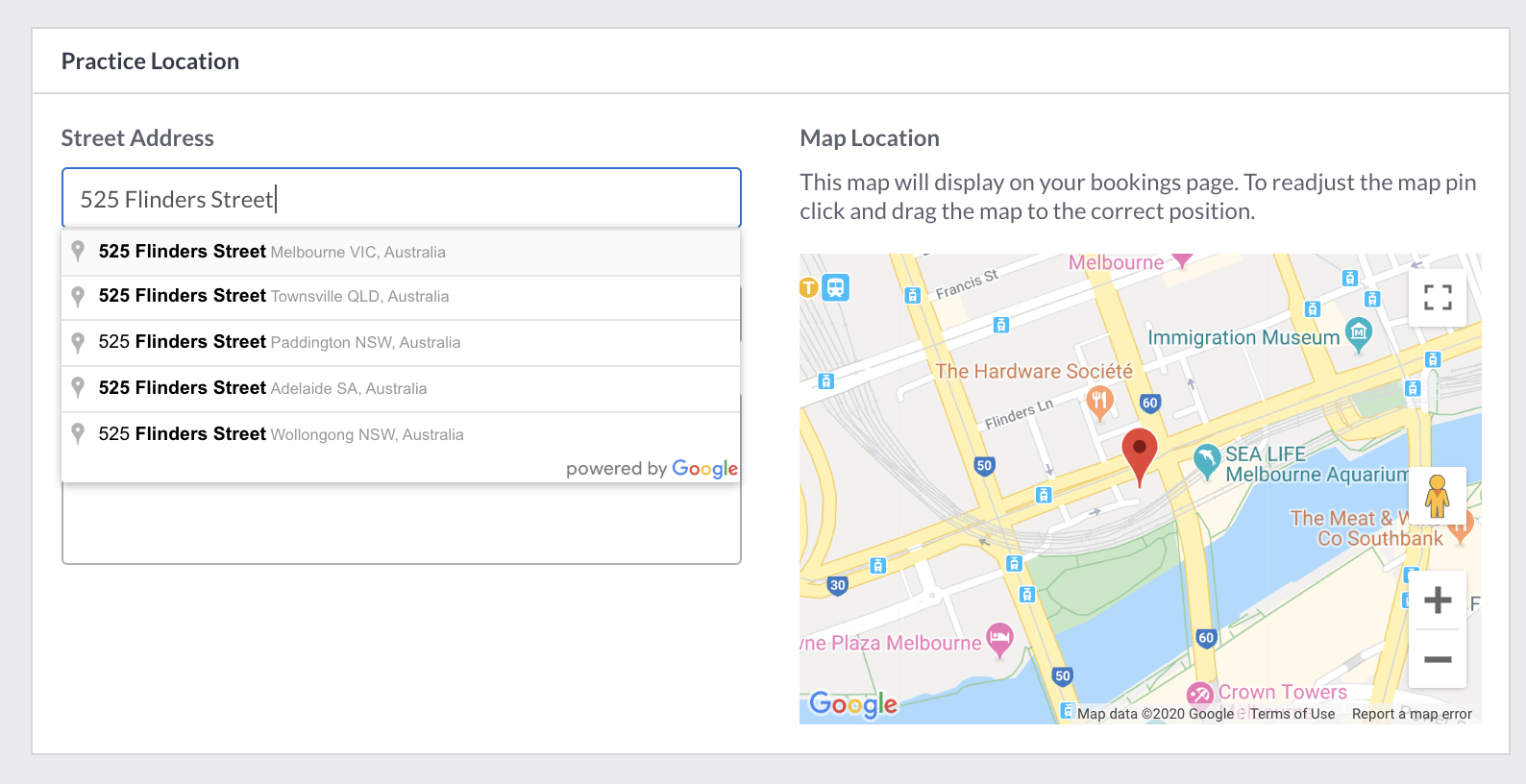The image depicts a detailed user interface of a basic map site. On the left side of the page, there's a search bar labeled "Street Address," where the user has typed in "525 Flinders Street." The main section of the interface on the right showcases a map view powered by Google Maps, as indicated by the Google logo at the bottom left corner of the map. The search results provide multiple location options within Australia, including cities like Melbourne and Adelaide. The highlighted location is in Melbourne, adjacent to prominent landmarks such as the Sea Life Melbourne Aquarium near a river that flows through the city. Other nearby points of interest include the Hardware Society and the Immigration Museum.

Above the map interface, there is an informative text box instructing users that the displayed map location will appear on their bookings page. It guides users to click and drag the map to adjust the pin to the correct position. Additionally, the map interface features the iconic outline of a person, which can be dragged onto the map to enable street view functionality.